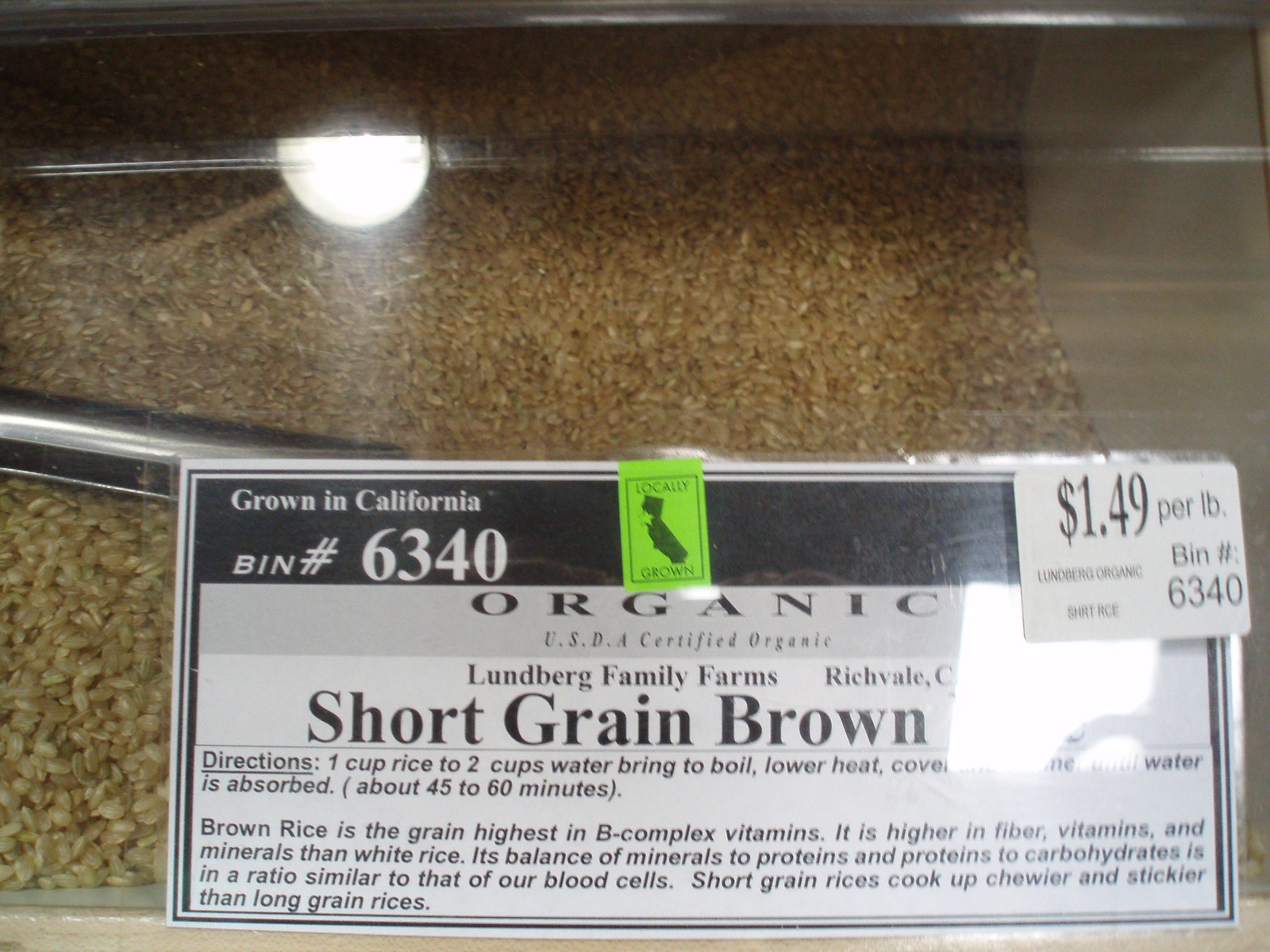This image features a detailed label for short grain brown rice, prominently displayed on a lime green sticker. The label provides clear cooking instructions: use one cup of rice with two cups of water, bring to a boil, and then cook for 45 to 60 minutes. It highlights that short grain brown rice is exceptionally high in B-complex vitamins and contains various beneficial minerals. The rice boasts a nutritional composition similar to that of human blood cells, enhancing its health benefits. Unlike long grain rice, this variety cooks up chewier and stickier. Additionally, the sticker proudly states that the rice is grown in California. Priced at $1.49 per pound, this rice is housed in a bulk bin, allowing customers to dispense the amount they need into their own bags, facilitated by a light above the bin for easy visibility.